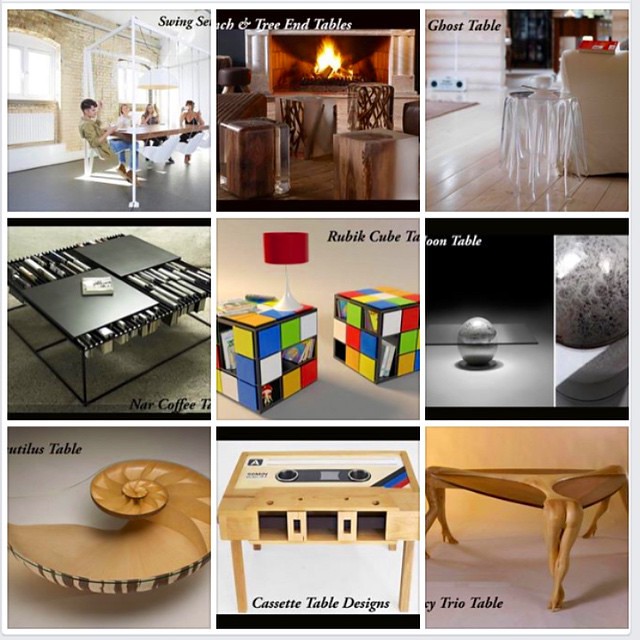This square image depicts a nine-item table catalog grid, with each cell showcasing distinct, avant-garde table designs. 

In the top-left cell, there’s an image of four people seated around a ‘Swing Set Table,’ where the tabletop is seemingly suspended, creating a floating illusion among swing-style seating. To its right, a contemporary room is presented with an airy ambience, featuring a fireplace alongside vertically standing rectangle tables. The top-right cell showcases the ‘Ghost Table,’ a clear, circular design with a couch in the background, characterized by its descending, transparent legs that evoke an ethereal feel.

The middle-left cell introduces the ‘NAR Coffee Table,’ a modern, pewter-colored square piece, functional yet stylish. Adjacent to it is a pair of innovative ‘Rubik’s Cube Side Tables,’ which mimic the colorful, multidimensional puzzle and come topped with a red-shaded, white-base lamp. The middle-right cell features a distinctive table with an egg-shaped marble base and a rectangular glass tabletop, exuding a sleek, artistic vibe.

In the bottom-left cell, a wooden table shaped to mimic the interior spirals of a conch shell stands out, demonstrating intricate craftsmanship. The centerpiece of the lower row is the ‘Cassette Table,’ designed to resemble a vintage audio cassette with specific areas to house small items. Finally, the bottom-right cell displays the ‘Trio Table,’ a triangular piece supported by legs sculpted to resemble human legs and buttocks, artistically provocative in nature.